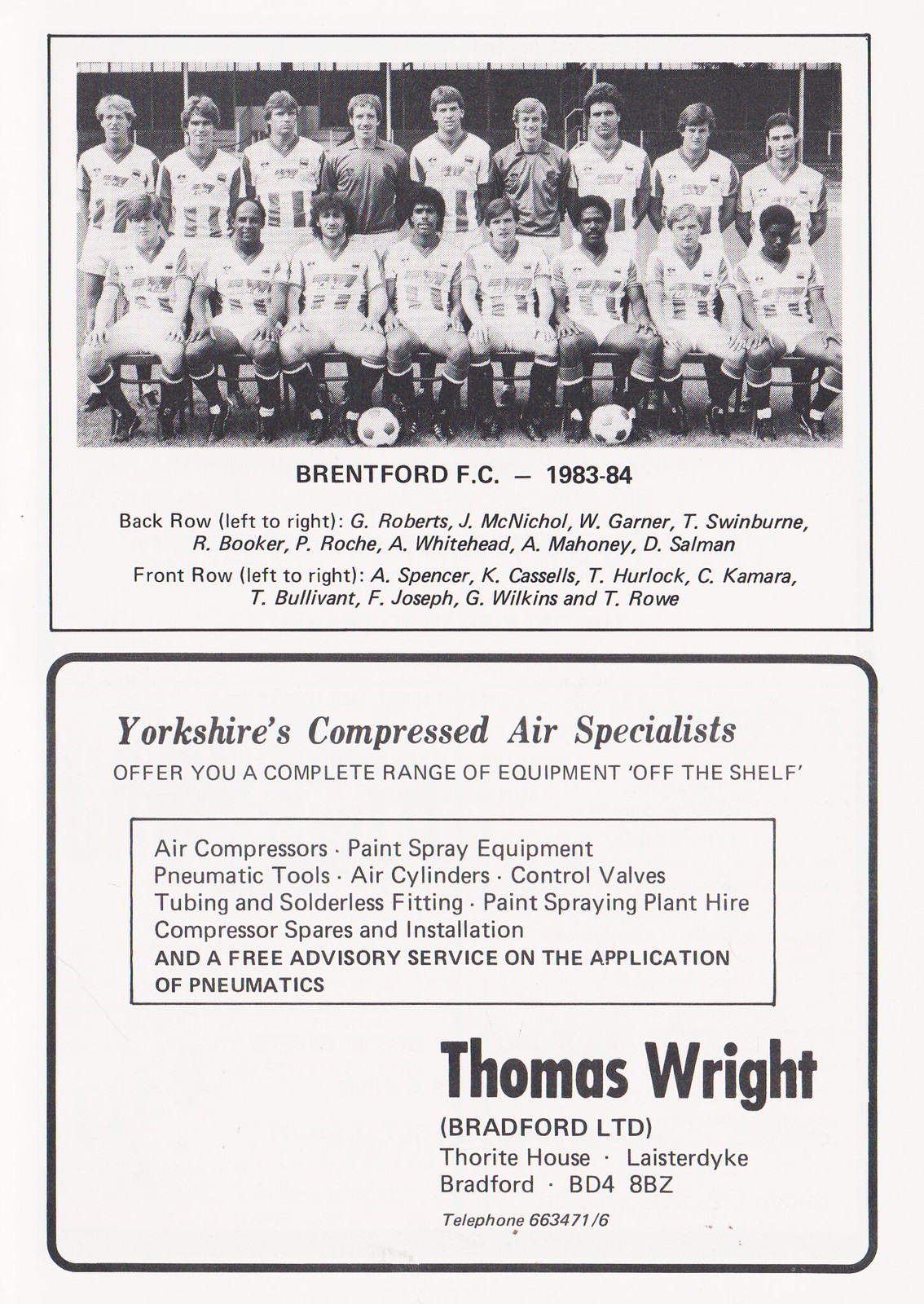The black-and-white image appears to be a vintage advertisement, likely from a newspaper or magazine, featuring Brentford FC from the 1983-1984 season. The top half of the image showcases a team photograph consisting of two rows of soccer players in uniform: the front row is seated on chairs, while the back row stands behind them. Their outfits are likely all white, and two soccer balls are placed on the grass in front of the group. Above the photo, the text identifies the team as "Brentford FC 1983-1984." Beneath the team photo, it lists the names of each player from left to right for both the back and front rows. 

The bottom half of the image serves as an advertisement for Yorkshire's Compressed Air Specialists, offering a complete range of equipment. The ad is framed with various details about the services provided by the company. In the lower right corner, the ad features the company name, "Thomas Wright Bradford Limited," along with its address and telephone number: Thor Wright House, Leicester Dyke, Bradford BD4 8BZ. This vintage assembly of imagery and text likely aimed to highlight team sponsorships, possibly for a yearbook or commemorative publication.